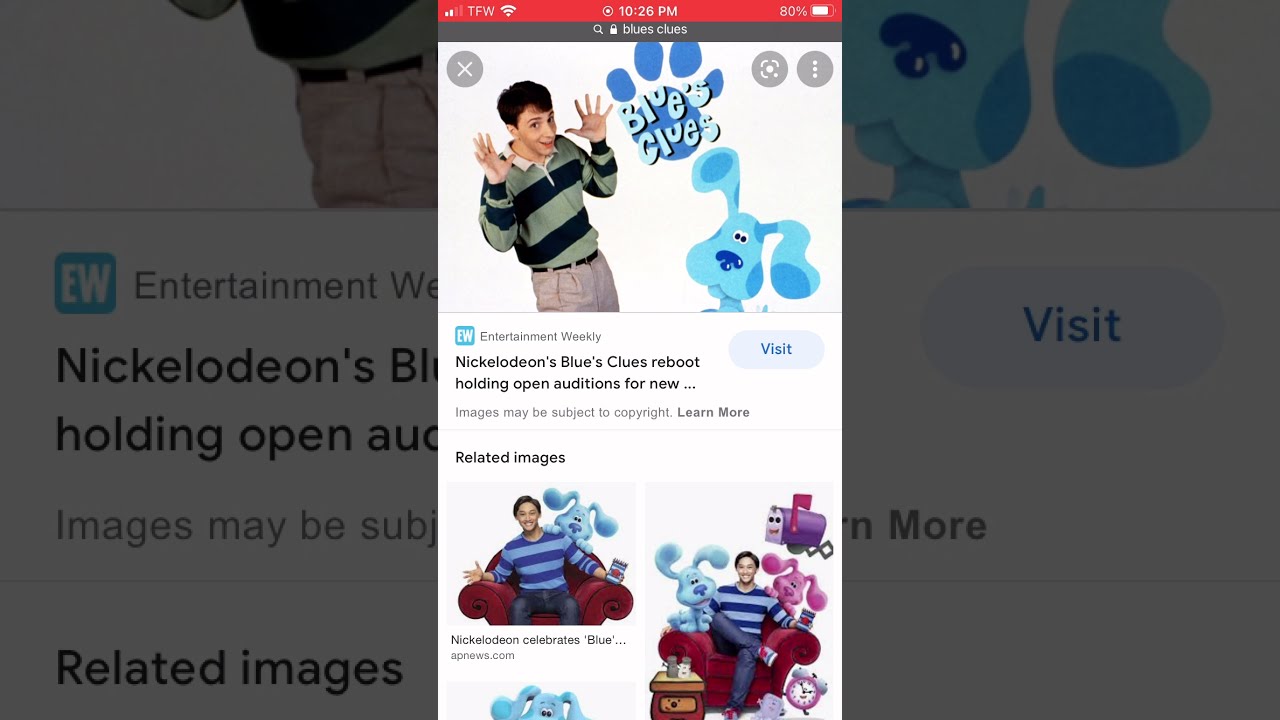The image displays a detailed screenshot from a smartphone at 10:26 PM with 80% battery, indicated by a top status bar featuring a Wi-Fi signal and a TFW logo. The main content is a Google search result for "Blue's Clues," showing an article from Entertainment Weekly about open auditions for Nickelodeon's Blue's Clues reboot. The top of the webpage features a man identified as Steve from Blue's Clues, wearing a long-sleeved shirt with black and green stripes, khakis, and holding his hands up with fingers spread wide. To the right of him is the Blue's Clues logo, a blue paw print with the text "Blue's Clues" in a lighter blue font. Below the logo, there's an animated image of Blue, the blue dog with darker blue spots, a big blue nose, and close-set eyes. The layout suggests it's a typical Google search result page, complete with a white background and a "Visit" button.